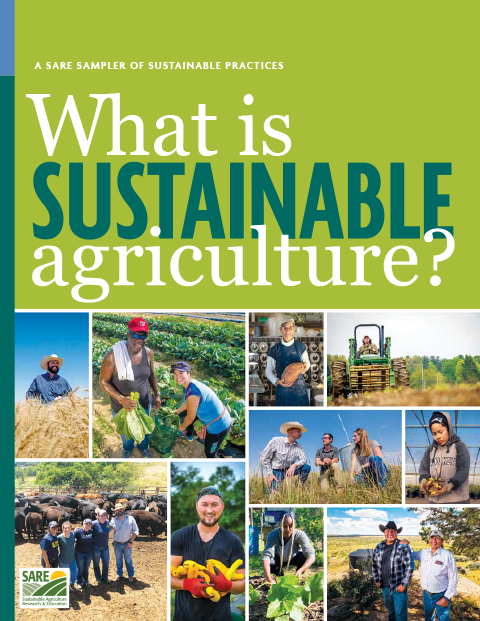The image is a vertical rectangular cover, potentially from a book, pamphlet, or document with a focus on sustainable agriculture. The cover features a slender dark green and light blue line on the left, simulating the edge or binding of a book. A large dark green horizontal rectangle dominates the top, containing the title in white and green typography: "A SARE Sampler of Sustainable Practices. What is Sustainable Agriculture?" Beneath this title, a neatly arranged grid displays 10 photographs, each bordered in white. These images depict various individuals, mostly adults, engaged in agricultural activities, smiling under the sun. Specific scenes include a man inspecting wheat, a couple standing by rows of lettuce, a person operating a tractor, and a man holding yellow squash. One photo shows two men, one in a cowboy hat and the other in a baseball cap, standing side by side with a field behind them. The collection of images illustrates diverse sustainable farming practices and aims to educate about sustainable agriculture.